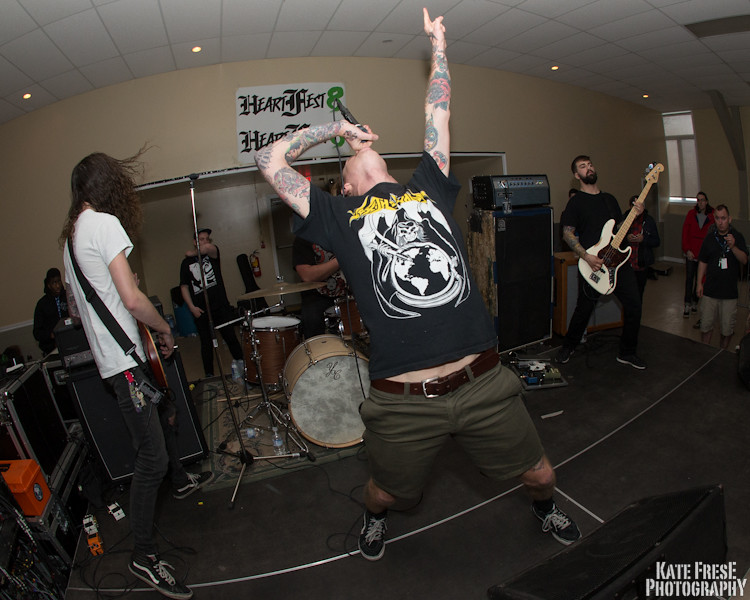The photograph depicts a heavy metal band performing on a platform that resembles a school auditorium. The lead singer stands at the center, passionately singing into a handheld microphone, with both arms raised and fingers pointing upward. His heavily tattooed arms are visible as he sports a black t-shirt featuring graphic designs like a skull and crossbones holding a dagger, and an image of the world, paired with shorts and sneakers. To his right is a bass guitarist, also tattooed and dressed in a black t-shirt and jeans. The guitarist to the left is in a white t-shirt, has very long hair and black jeans, and is playing with his back turned to the audience. Standing behind them is a drummer. The backdrop prominently displays banners reading "Heart Fest 8." The audience includes several individuals wearing name tags on straps, suggesting it may be at a concert or convention. Additional personnel and equipment, such as speakers and double doors, are also visible in the background. The photograph is credited to Kate Fress Photography in the lower right corner.